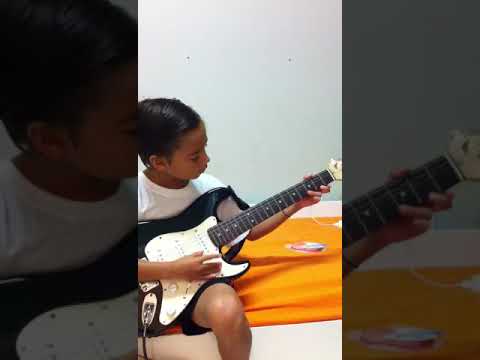This photograph captures a focused young boy, approximately 10-12 years old with short, combed black hair and dark brown skin, possibly of South Asian descent. He sits cross-legged on a bed covered with an orange sheet, situated in a room with a white wall backdrop. Dressed in a white T-shirt and black shorts, he meticulously strums a black and white electric guitar with a maple-colored headstock. The guitar, which is plugged in, rests on his lap as he uses his right hand to play the strings and his left hand on the fretboard. His intent gaze is fixated on the guitar, indicating he's deeply engaged in practicing. The photograph appears vertically cropped and might have been taken with a smartphone, featuring blurred and stretched versions of the original image on the sides. Though the background wall appears dull due to lighting, the focus remains on the boy and his instrument. Additional objects are scattered on the bed, suggesting a casual indoor setting.